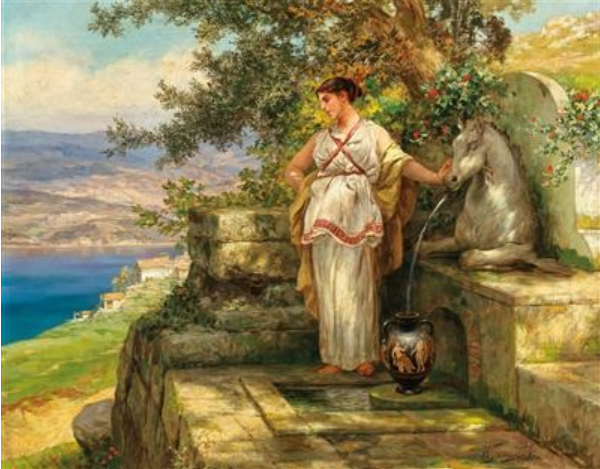In this vibrant and detailed painting, a woman dressed in a flowing white gown with yellow fabric flowing behind her stands at a fountain, sculpted in the form of a horse's head and front hooves. Water gushes from the horse's mouth into a black urn adorned with images of people, which she has placed on a tiled, brick-like area below the sculpture. The woman possesses short, dark brown hair and gazes downward towards the water, seemingly lost in thought. In the background, a serene blue body of water, resembling a lake or ocean, stretches out to the left, bordered by a tree with lush, cascading leaves behind her. Further still, a range of mountains and scattered clouds paint a picturesque horizon, indicative of a well-established ancient Greek setting. The scene, filled with classical elegance, also features various details such as additional houses, a hint of a city nearby, and flowers sprouting behind the horse fountain, enhancing the overall atmosphere of a tranquil yet sophisticated landscape. The woman stands on a marble platform that resembles the entrance to a grand structure, adding to the sense of antiquity and civilization.